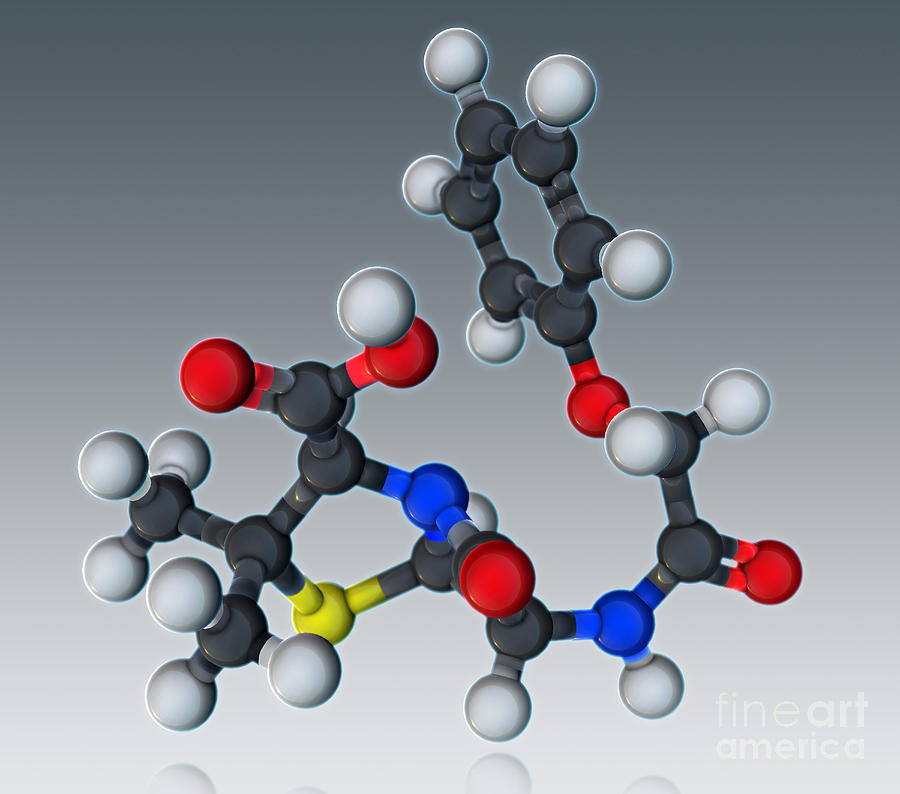This scientific diagram showcases a complex molecular structure composed of various interconnected spherical molecules in vivid colors, including white, black, red, blue, and yellow. The spheres are arranged into distinct patterns such as hexagons and pentagons, hinting at cyclic aromatic structures, possibly depicting a sequence in a DNA chain. Each sphere likely represents different atoms, with whites possibly being hydrogen, reds for oxygen, blues for nitrogen, and yellow for sulfur or phosphorus. The molecules are connected with stick-like bonds, forming intricate shapes that highlight the assembly. The background features a grayish-black gradient, emphasizing the vibrant molecular arrangement. Notably, the image includes a caption that reads "Fine Art America" in the bottom right corner.